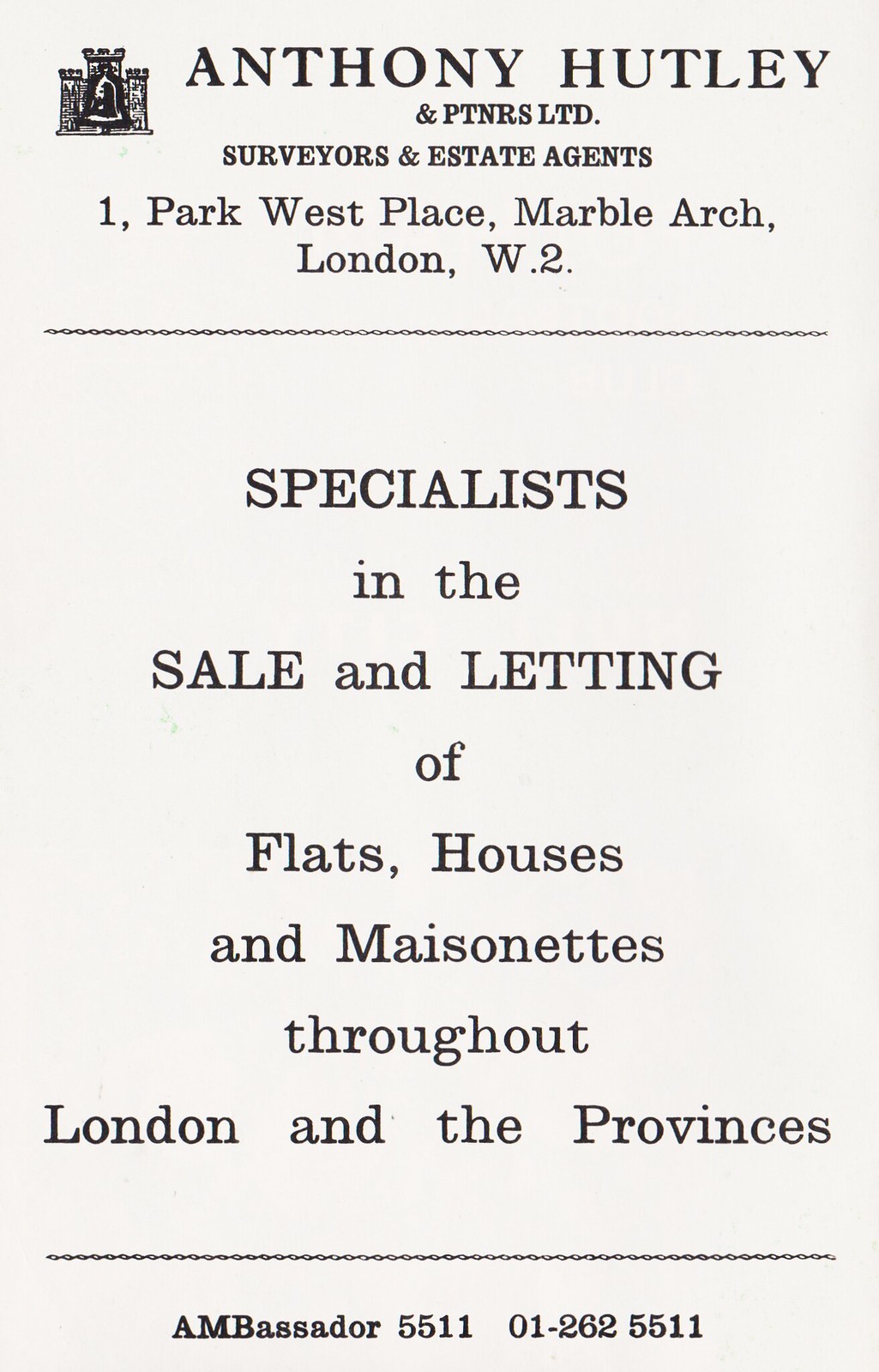The image depicts an old business card printed on white paper with black text. At the top left corner, there is a small crest resembling a castle. The card prominently features the name "Anthony Hutley and Partners Limited, Surveyors and Estate Agents." It lists the address as "1 Park West Place, Marble Arch, London, W2." Beneath this, the card emphasizes in capital letters: "Specialists in the Sale and Letting of Flats, Houses, and Maisonettes throughout London and the Provinces." At the bottom, contact details are provided: "Ambassador 5511, 01-262-5511." The design is quite minimalist, featuring only black print on a white background.